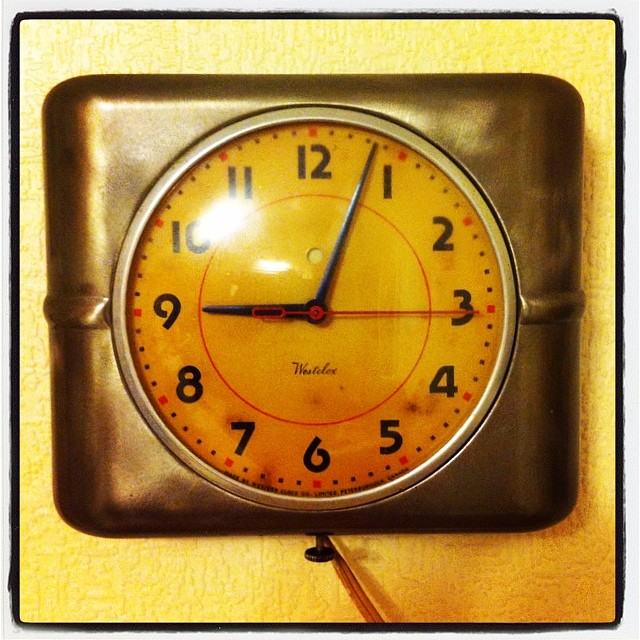This photograph captures the remnants of what seems to be a vintage folding travel clock. The clock is encased in a yellow square container with a distinct black border. At the center of this container lies a recessed metallic bezel holding the clock face, which is positioned on the right side. The clock stem is at the bottom of the image. The once-white clock face now has an antique, yellowish-orange patina. It features simple black numerals ranging from 1 to 12, encircled by a red ring beneath the numbers. The black hour and minute hands, along with a red seconds hand, indicate the time as just past 9:03. The overall worn appearance suggests the clock has seen significant use over the years.